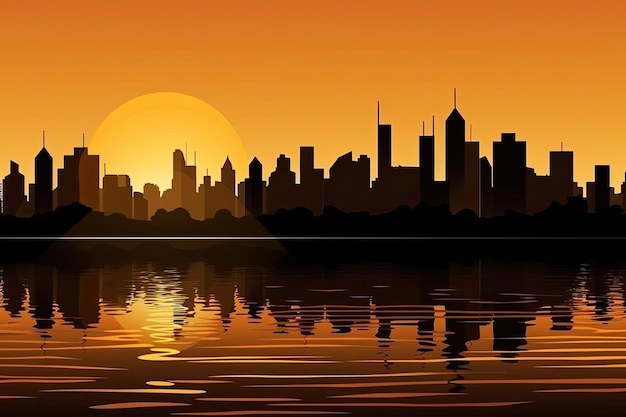This digital illustration depicts a city skyline during sunset, showcasing a series of high-rises and skyscrapers in sharp silhouette against a striking, orange-hued sky. The setting sun, positioned on the left, is a large yellow orb with a white center, partly obscured by the buildings. In the foreground, a body of water mirrors the entire cityscape, displaying the skyline's reflection with slight ripples that add a dynamic distortion. The water's surface is notably shiny, enhancing the vividness of this mirrored image. The artwork is text-free, focusing solely on the serene yet dramatic interplay between the silhouetted skyline and its reflected image in the glowing, rippling water.